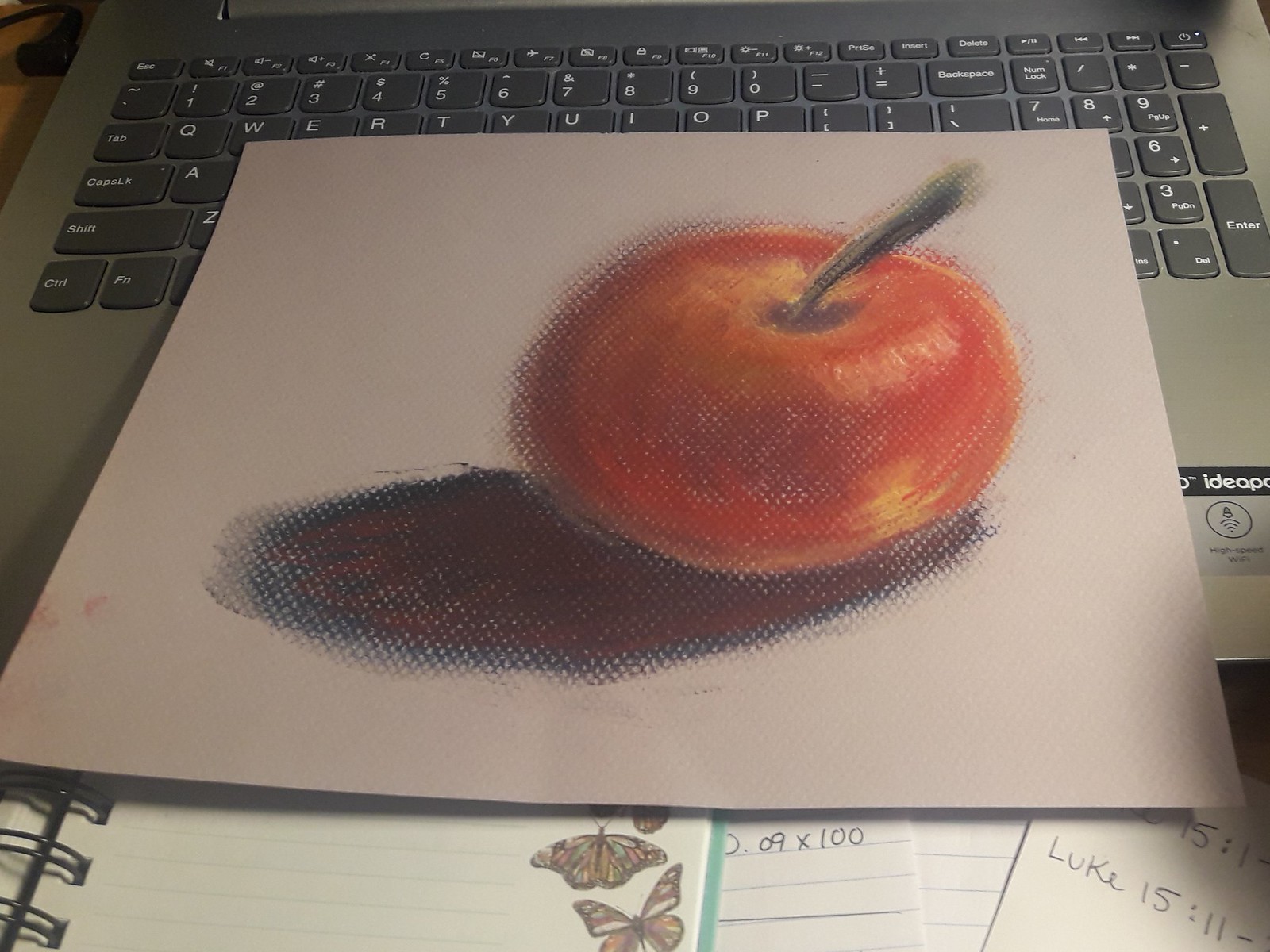A detailed real-life photo showcasing a textured, square piece of paper displaying a meticulously crafted hand-drawn illustration of a fruit, potentially an apple. The artwork boasts a variety of red hues, suggesting the use of pastels or a rough painting technique, and features a glare and dark spots that contribute to its realistic appearance. The apple's edges appear fuzzy, and it has an oversized stem rendered in dark tones like black and gray. Beneath the apple is a pronounced black shadow intermixed with some red hues. Two smudges are visible on the left side of the paper. Surrounding the central illustration, the lower section of the frame captures assorted handwritten notes and an open spiral-bound notebook adorned with butterfly icons and lines, as well as a reference to Luke 15:11. The upper half of the image, beneath the artwork, reveals part of a laptop keyboard with black keys bearing white letters and a silver frame. A sticker reading "IdeaP" with an accompanying logo is also visible on the laptop.